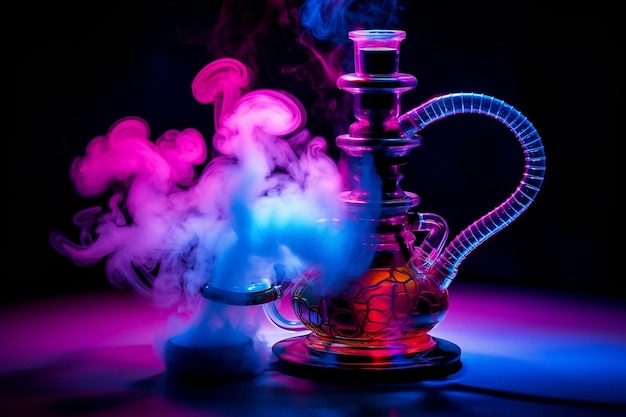This close-up photograph captures an elaborate glass bong set against a completely black background, accentuating its vivid colors and intricate details. The brightly colored bong features a unique design reminiscent of a whimsical science experiment or mystical apparatus. The bong has a complex structure with cylindrical sections separated by flat discs, tapering into shapes that widen and narrow, ending in a rounded, genie's lamp-like base that sits atop a wide glass disc. A prominent glass hose curves from the top to the base of the bong.

The bong is adorned with a stained-glass appearance towards the bottom, giving it a mosaic-like texture. The top piece of the bong showcases accents of black and purple, illuminated by nearby lighting, reflecting hues of red, purple, blue, and pink. Smoke billows from the bong, beginning as neon blue and transitioning through shades of pink and purple, creating an eye-catching and colorful display. The surface beneath the bong refracts more of this vivid color, with reflections showing hues of pink, blue, and gray.

Overall, the photograph presents an aesthetic interplay of colorful smoke and glass, capturing a mesmerizing and dynamic scene that is both fun and intriguing.